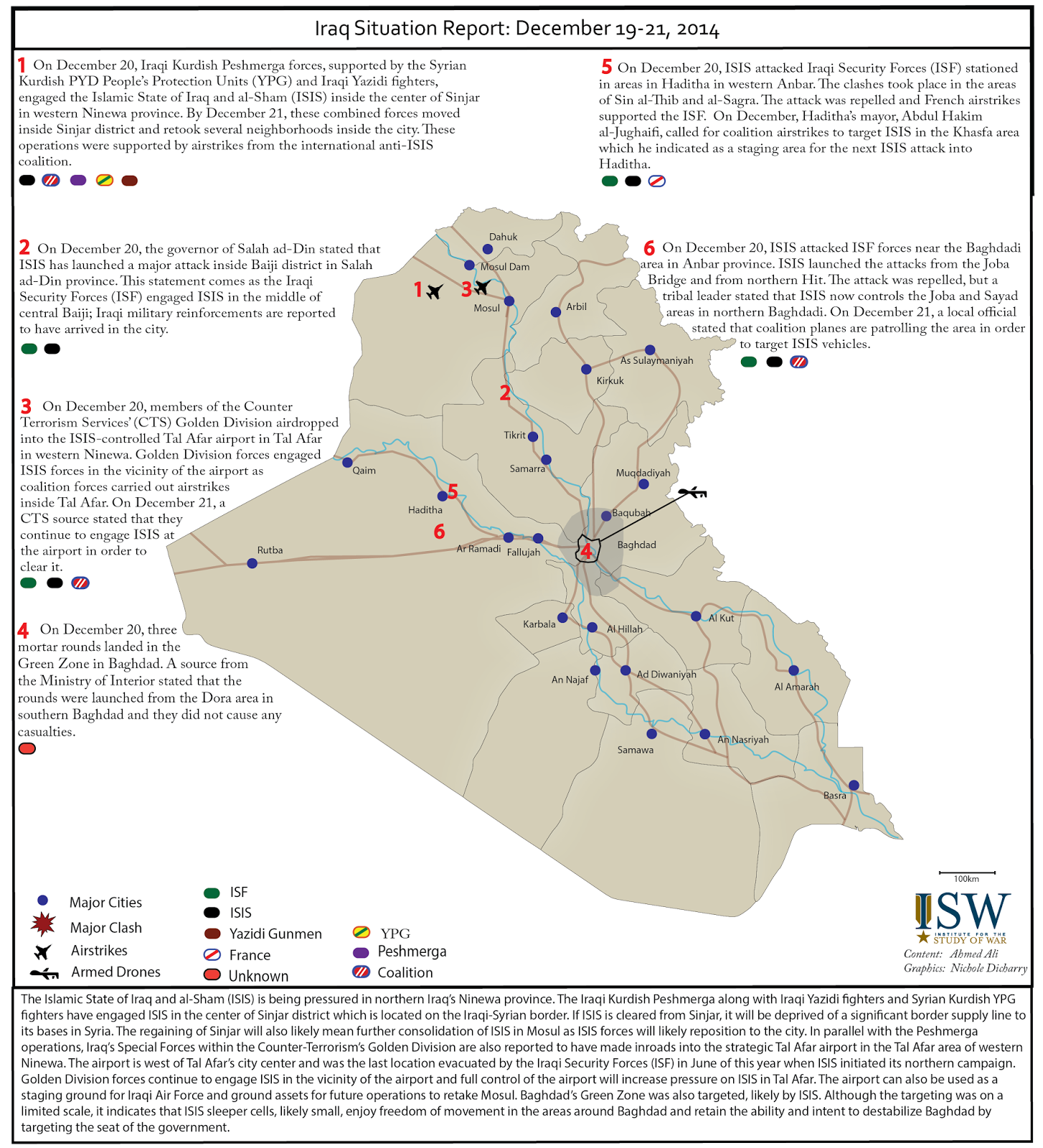This image is a beige-colored map depicting Iraq, focusing on the country's situation report from December 19th to 21st, 2014. The map features various cities clearly labeled, with key locations marked by airplane icons indicating airports. Among the cities, you can spot places like Bajij.

The map is annotated with numbered indicators from one to six, each corresponding to different military actions and events that took place during the specified dates. For example, note one highlights that on December 20th, Iraqi forces, supported by Syrian People's Units and other allies, undertook certain operations. Although the report mentions the period from the 19th to the 21st, most noted actions within the map are concentrated on December 20th.

A legend at the bottom of the map uses various symbols to denote specific events and locations; for instance, a red icon represents a major clash. This detailed legend helps the viewer quickly interpret the significant aspects of military movements and key occurrences during the specified time frame. Overall, this map provides a concise visual summary of the strategic military events in Iraq over these three critical days in December 2014.